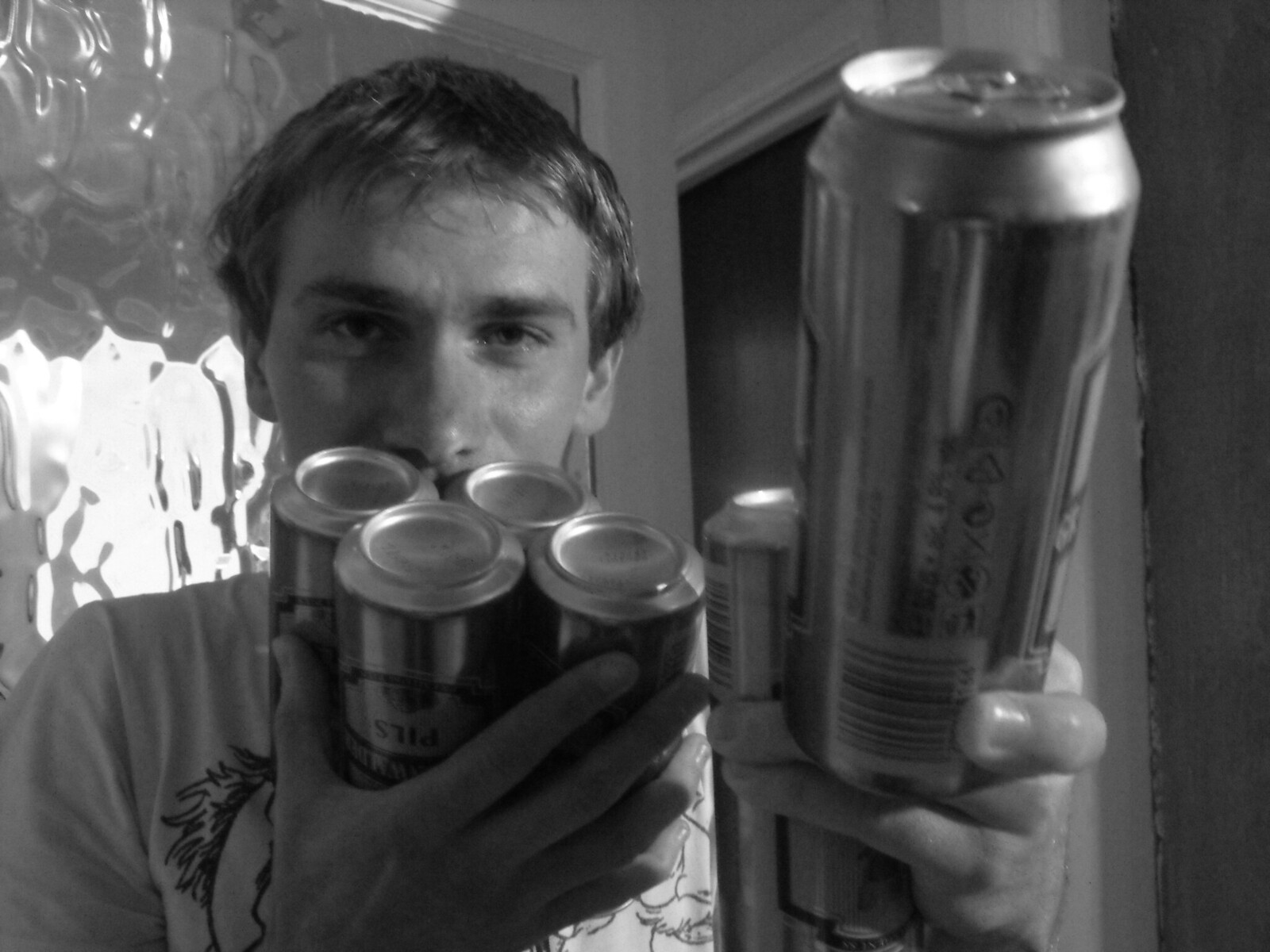In this black-and-white photograph, a young man of around 25 with short, light-colored hair stands indoors holding six large cans of Pilsner beer. He is wearing a graphic tee with a line drawing on it. Four of the cans are turned upside down and pressed against his mouth with his right hand, while the other two cans are held upright in his left hand towards the photographer. The man's eyes suggest he is smiling as he stares directly at the camera. Behind him, there's a patterned glass panel, possibly part of a door, and to his right, there is a doorway leading to a dimly lit passage. The image has an older, nostalgic quality due to its black-and-white format.